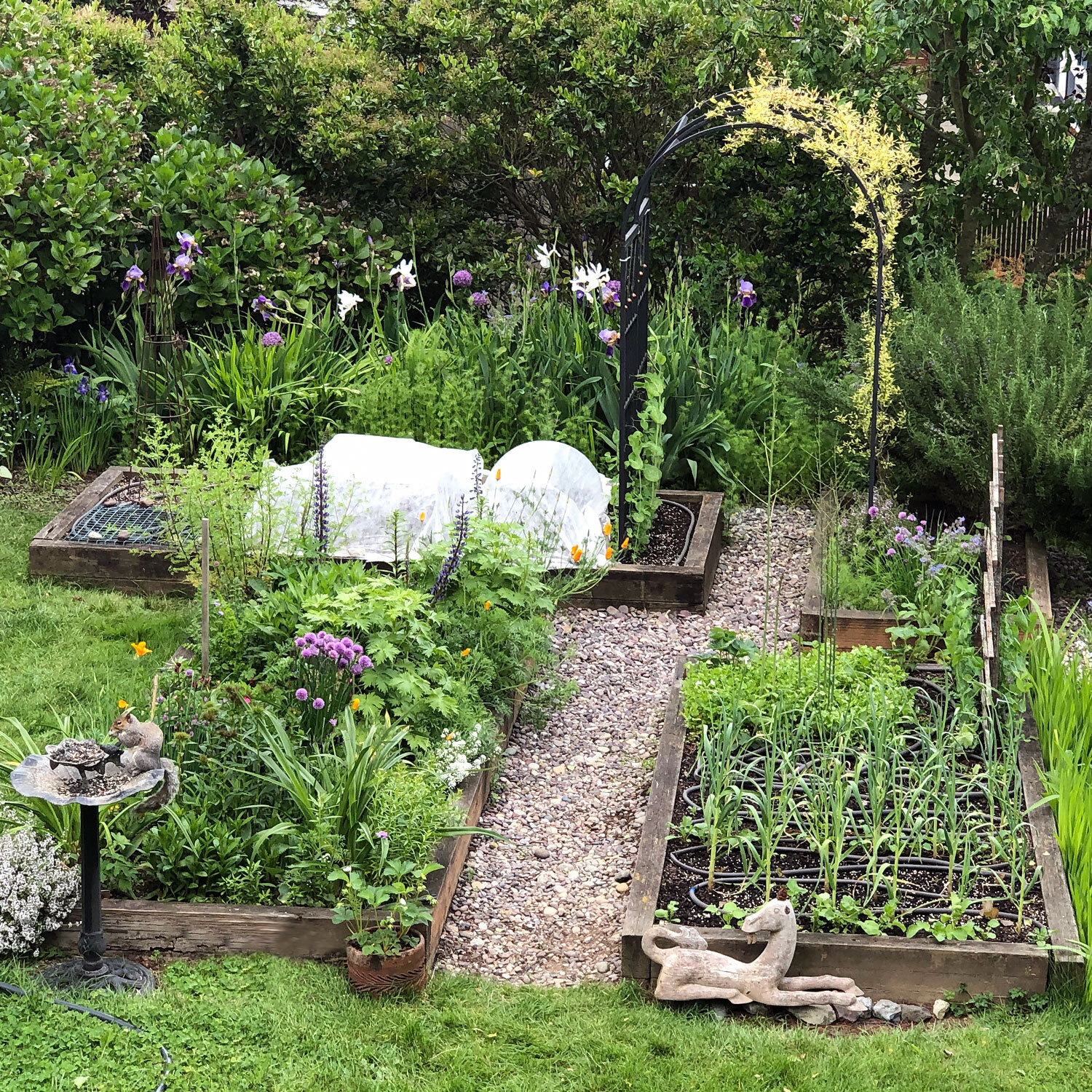The photograph showcases a meticulously maintained garden featuring a lush carpet of green grass, albeit slightly overgrown. At the center of the scene are raised beds, bordered by wooden boundaries, where various plants flourish, nearly all adorned with verdant leaves. Interspersed among these plants, some of which extend taller while others remain shorter, are colorful flowers, primarily purple and occasionally yellow or white. Small grey rocks and pebbles form a neat walkway between the beds. At the back, a charming arrangement of trees with green leaves rises behind the flowering plants. A birdbath—currently occupied by a squirrel—adds a whimsical touch along with a nearby sculpture. Some plants appear to be covered with white cloth for protection. Notably, there are structures that seem to be cages, possibly for supporting tomato plants, and an assortment of herbs including what looks like chives and lavender, making this garden both vibrant and well-nourished.